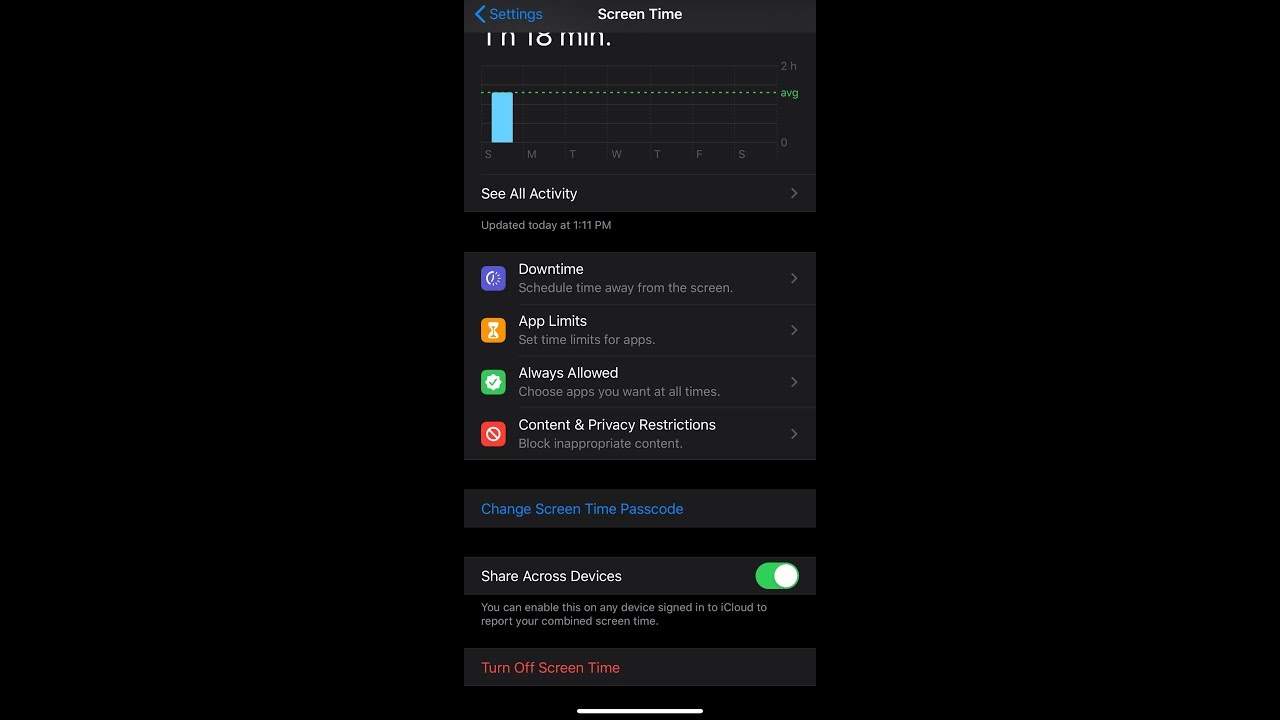This detailed screenshot of an iPhone, configured with dark mode, displays the "Screen Time" settings. The black background emphasizes various controls and options, including "Downtime," "App Limits," "Always Allowed," and "Content & Privacy Restrictions." A prominent red option labeled "Turn Off Screen Time" catches the eye. The settings screen features the typical layout and design of iOS, with a back button labeled "Settings" at the top left, confirming its iPhone origin. The dark theme enhances readability and reduces eye strain, offering a sleek and modern user interface.